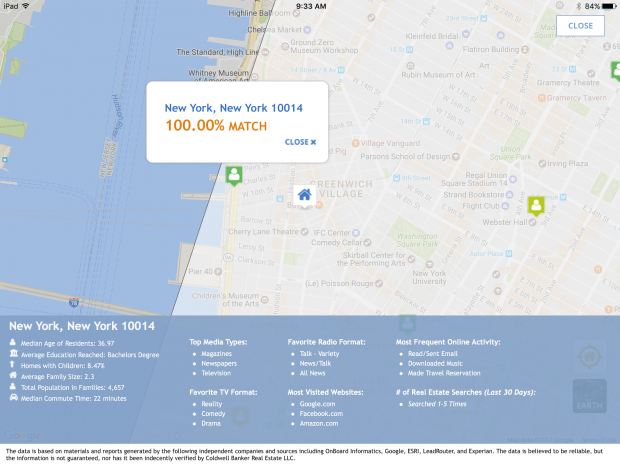**Descriptive Caption:**

This image is a detailed screencap of a map depicting a section of western New York, likely taken on an iPad. The map uses standard cartographic colors with blue representing the ocean, and green, brown, and gray illustrating different land areas. White lines crisply delineate the streets. A semi-transparent white boundary outlines the map, particularly noticeable on the right side.

A pop-up within the map highlights "New York, New York 10014" with a 100.00% match and offers a link to close the pop-up, denoted by a small 'X' icon. The map also features various icons: three green pin markers with head-and-shoulder profiles, differentiated by shades of green, and a blue house icon. 

At the bottom, within a blue text block, more information reads "New York, New York 10014" accompanied by census data and details about top neighborhood favorites. The iPad's status bar shows the time at 9:33 AM with the battery at 84% charge.